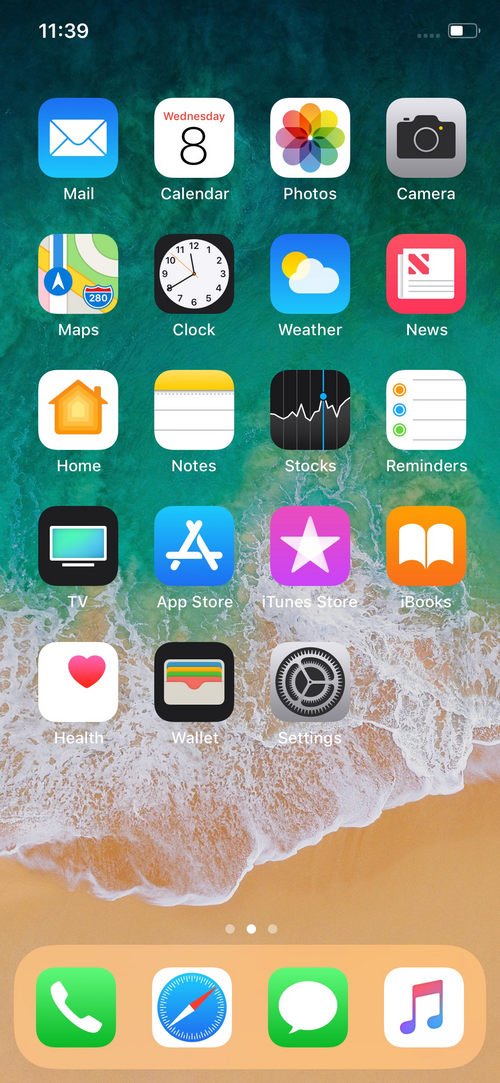This screenshot captures the home screen of a smartphone, instantly recognizable by the arrangement of app icons and the status bar. At the top left of the screen, the carrier information shows "AT&T" with a 4G connection. Centered at the top, the time is displayed as 4:35 PM. On the top right, the battery icon indicates it is currently charging, denoted by a lightning bolt symbol, with the charge nearly full.

The home screen is populated with various apps. The first app in the top left corner is the Mail app, which displays a red notification badge with the number 8, indicating there are eight unread emails. Other visible apps include Calendar, Photos, Camera, Maps, Clock, Weather, News, Home, Notes, Reminders, TV, App Store, iTunes Store, iBooks, Health, Waze, and Settings. 

At the bottom dock of the screen are four frequently used apps: Phone, Safari, Messages, and Music, arranged from left to right. 

The background image features a serene beach scene with gentle waves washing onto a smooth shore, exuding a calm, natural ambiance.